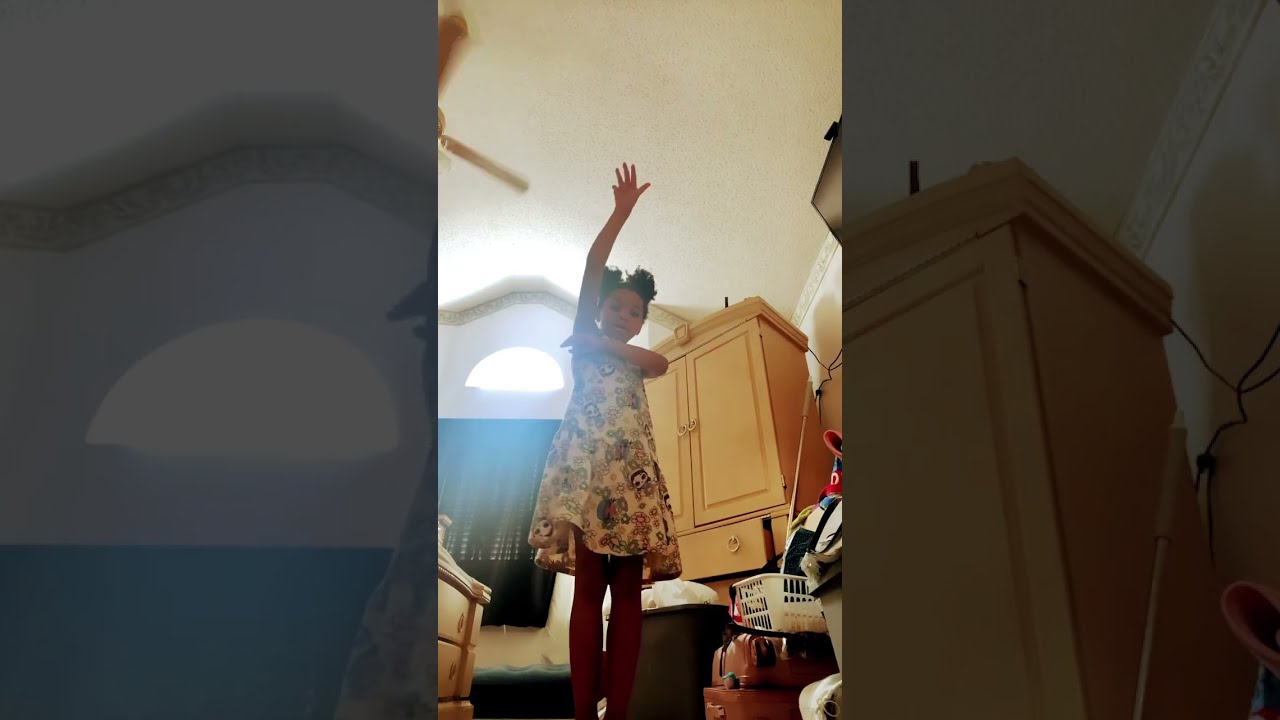The rectangular image is divided into three horizontal panels. The left panel is darkened, featuring a window with visible wall sections above and below it. The middle panel, brightly lit and seemingly superimposed over the larger image, showcases a young girl with short black hair facing the viewer. She wears a white dress with brown designs and has her right arm raised while her left arm crosses her chest. Behind her, to our left, is a window partially covered by a black curtain, with bright sunlight streaming through. To our right in the background, there's a tan-colored cabinet or armoire, and below it, various items such as a basket and other miscellaneous storage, suggesting a cluttered room. The right panel, also darkened, focuses closely on the right side of the cabinet seen in the middle panel and reveals some wires and part of the ceiling. Additionally, there is a touch of color from the girl's dress peeking in from the right edge of the image in the background panel. The overall setting is a well-lit room filled with various household items, indicating the scene is captured during the day.